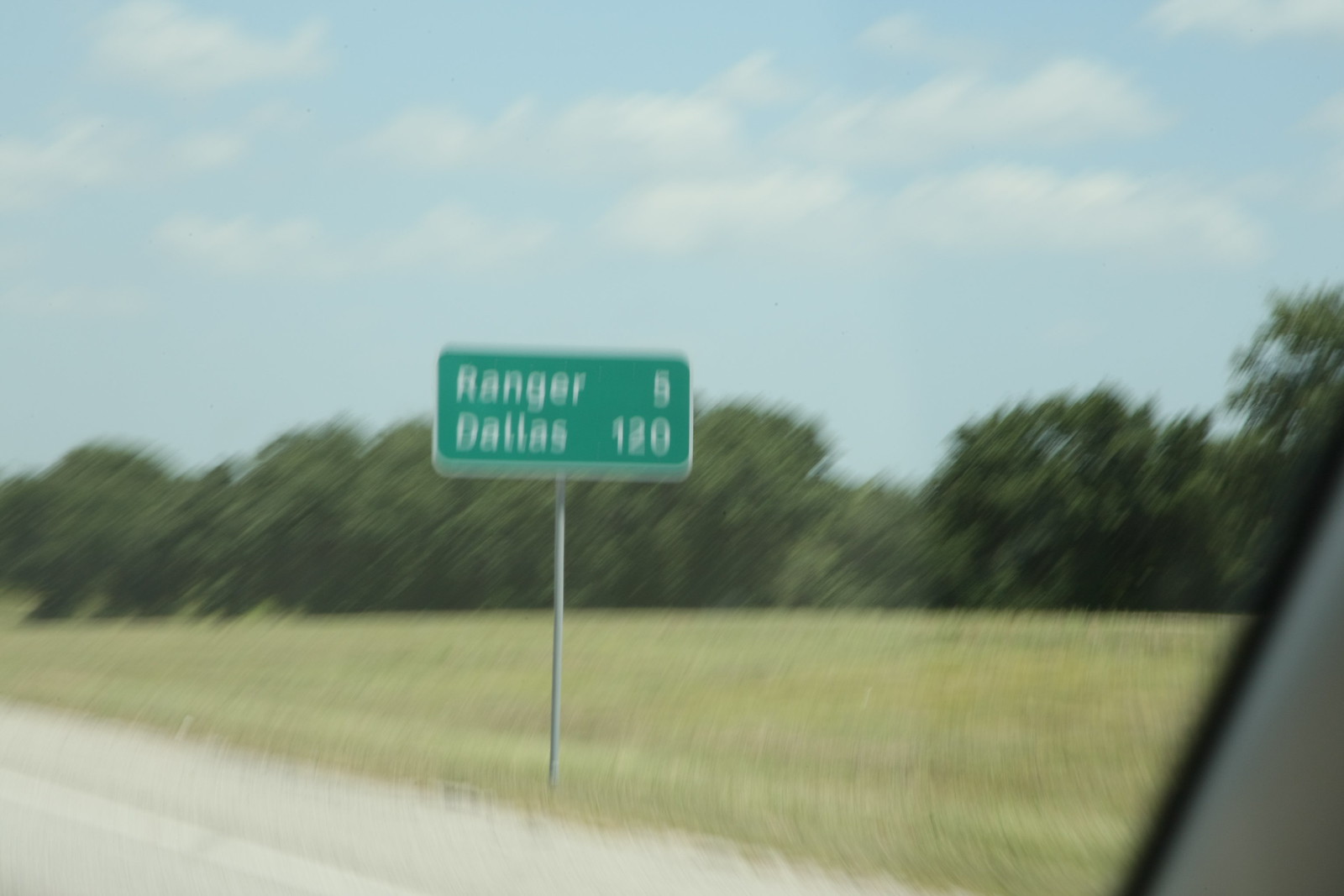A blurry horizontal photograph captures a green rectangular road sign, taken from within a moving car. The sign, featuring white text, indicates "Ranger 5 miles" and "Dallas 120 miles." This milestone marker stands against a backdrop of flat terrain dotted with dry grass in the foreground and a distant grove of trees. The partly cloudy sky suggests a hot day with heavy white clouds scattered across a blue expanse. In the bottom right corner, a small part of the car's gray interior and black weather stripping is visible, subtly framing the scene.